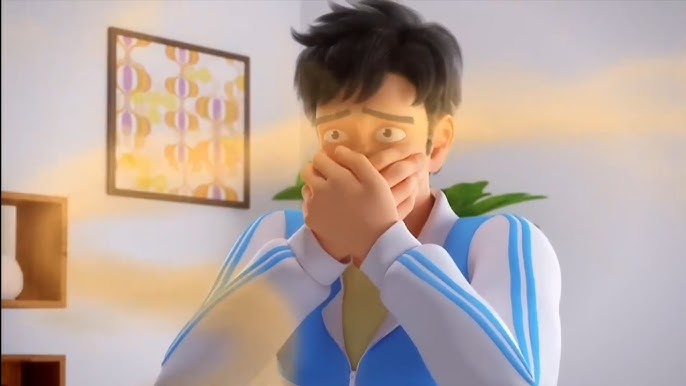This three-dimensional cartoon features a male figure, captured from just below the chest upward, centrally framed inside what appears to be a home. The man is wearing a white tracksuit with blue edging over a khaki shirt. His short, messy black hair almost touches his sharply drawn, expressive eyebrows that convey a sense of horror and disgust. His eyes, wide and perturbed, add to the emotional intensity of the scene.

He has both hands overlapping and covering his nose and mouth, suggesting he is reacting to a foul odor. This is further accentuated by a faint trail of brown gas depicted crossing from his body, implying he has just released a particularly unpleasant fart.

In the background, a simple indoor setting is portrayed: a blank wall transitions into a corner where a tiny shelf with a white vase is partially visible on the left, accompanied by a green plant. Additionally, a small abstract picture featuring possible flowers or orange and purple circular designs hangs on the wall. The overall impression is one of immediate, visceral reaction to a comically intense smell in a mundane domestic environment.